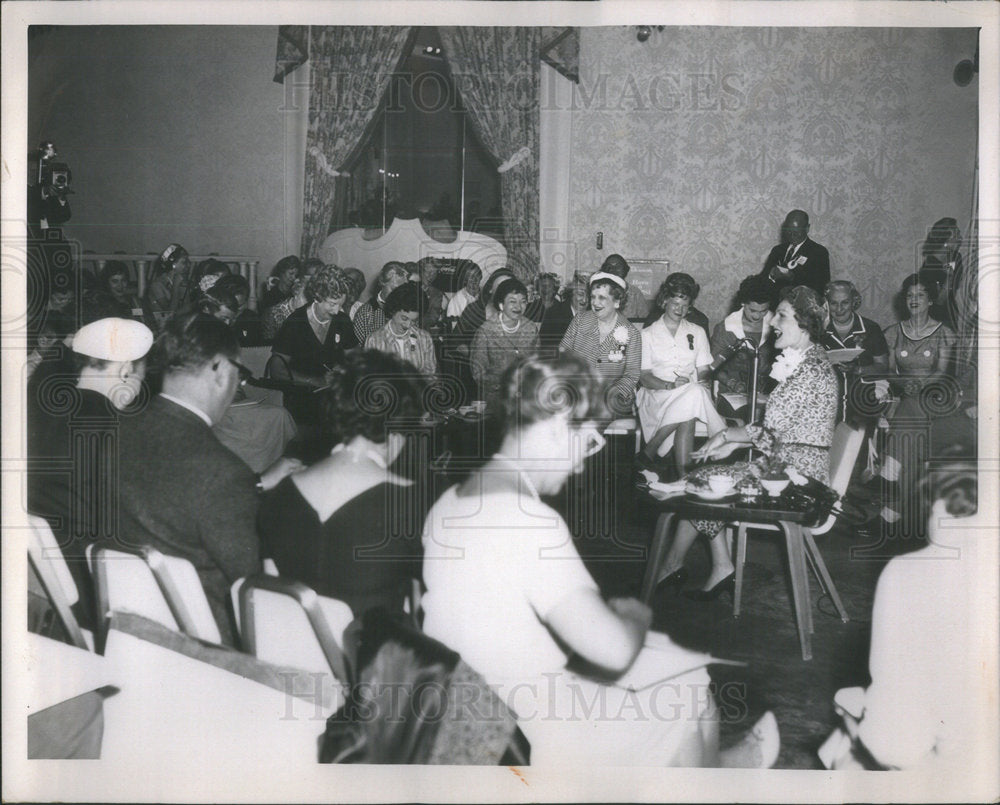This detailed black-and-white photograph, likely taken in the 1950s, showcases a group of people gathered at what appears to be an event. The background features a wall adorned with a patterned wallpaper, though the exact design is indistinguishable due to the monochrome nature of the image. In this setting, two rows of people are seated in chairs, with the first row featuring individuals with their heads bowed, possibly reading or following along with the event. In contrast, the individuals in the back row are engaged, smiling, and talking. A notable figure in profile is positioned between these rows. This woman, who is smiling and speaking, seems to be addressing the group and might be holding a microphone. The crowd, consisting mainly of middle-aged women dressed in 1950s-style dresses and hats, and a few men in suits, forms a half-circle around her. The photograph captures the essence of a historical moment, with the text "historical images" hinting at its significance. A man in the back right, possibly a sailor, is looking down, taking notes. The room's window is adorned with substantial draperies, adding to the period-accurate ambiance.